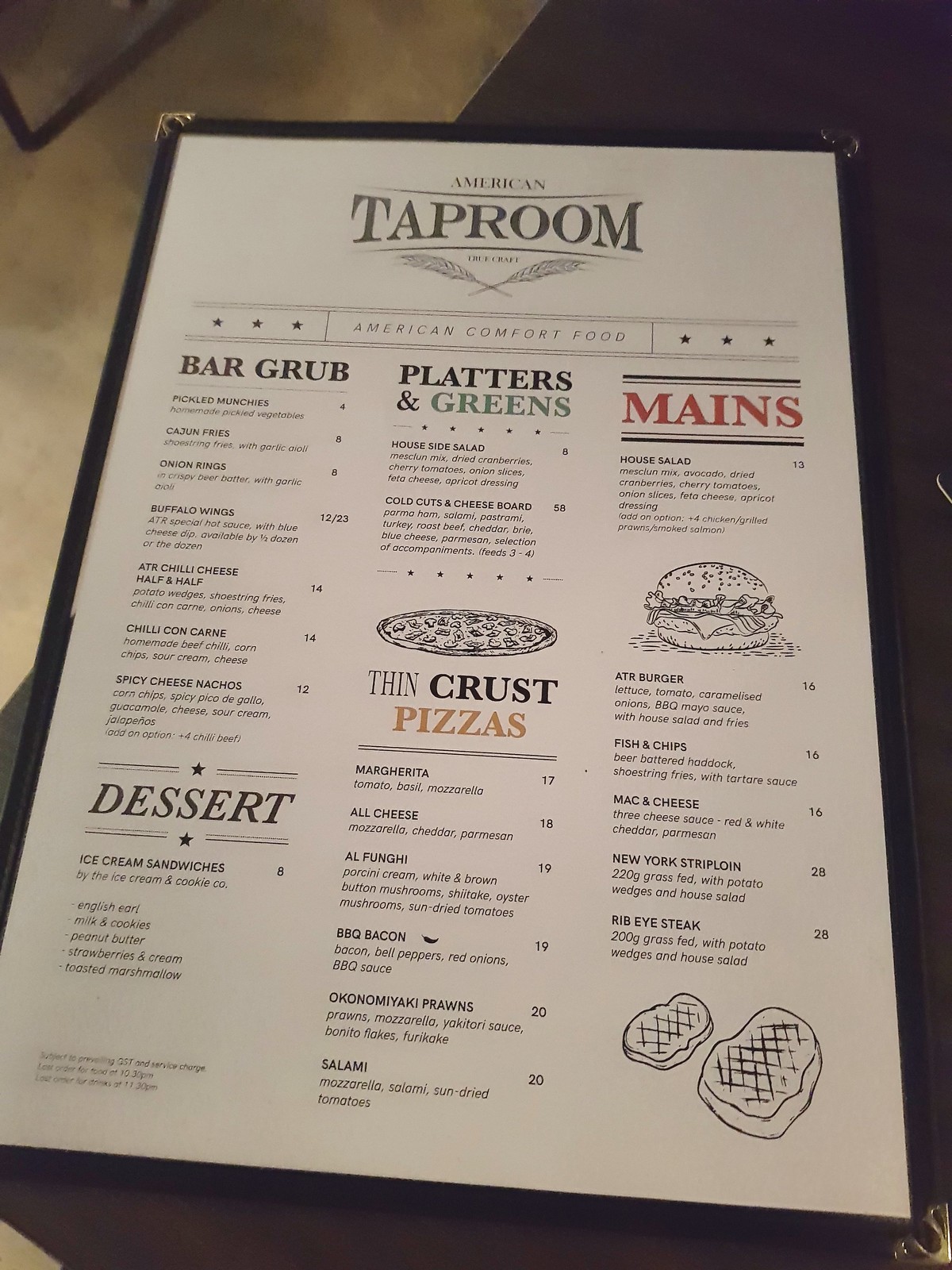This is a detailed description of a photo depicting a menu. The title "Taproom," specifically "America's Taproom," is prominently displayed at the top. On the left side, the menu is categorized under "Bar Grub," listing items such as Pickled Munchies, Cajun Fries, Onion Rings, Chili Corn Carne, and Spicy Cheese Nachos. Following that are the categories "Desserts," "Platters," and "Greens," each offering various selections. Centrally positioned on the menu is an illustration of a mini pizza, aligned perfectly with the spacing between the other subheaders. Underneath this, the category "Thin Crust Pizzas" is mentioned, detailing different pizza varieties. The next category is "Mains," and nearby is a drawing of a hamburger. Further down, towards the bottom right corner of the menu, there are illustrations of two steaks.